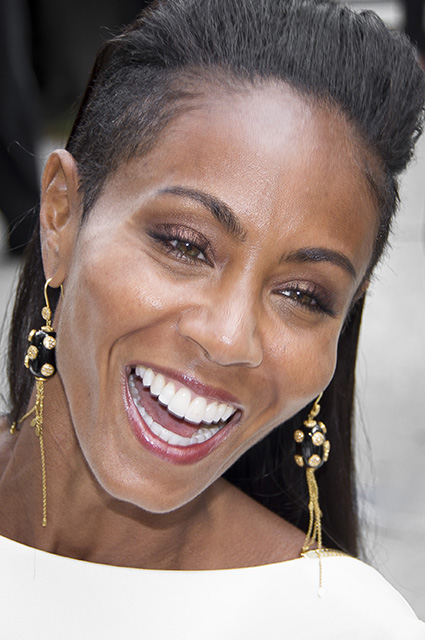This striking image is a very close-up shot of an African-American woman, centered in the frame, with a blurred background that is indistinguishable. The focus highlights her beaming smile, displaying her big white teeth. The woman wears large, elaborate gold earrings adorned with black balls and long, stringy gold chains. Her black hair is styled, pulled back, and sticking straight up, with a portion cascading down to the side. She sports a white top, and her face is brightly lit, enhancing her lipstick and eye makeup. The photograph captures her looking slightly down and to the side, surrounded by a backdrop of white and shades of gray, making her vibrant expression and detailed features the focal point of the image.